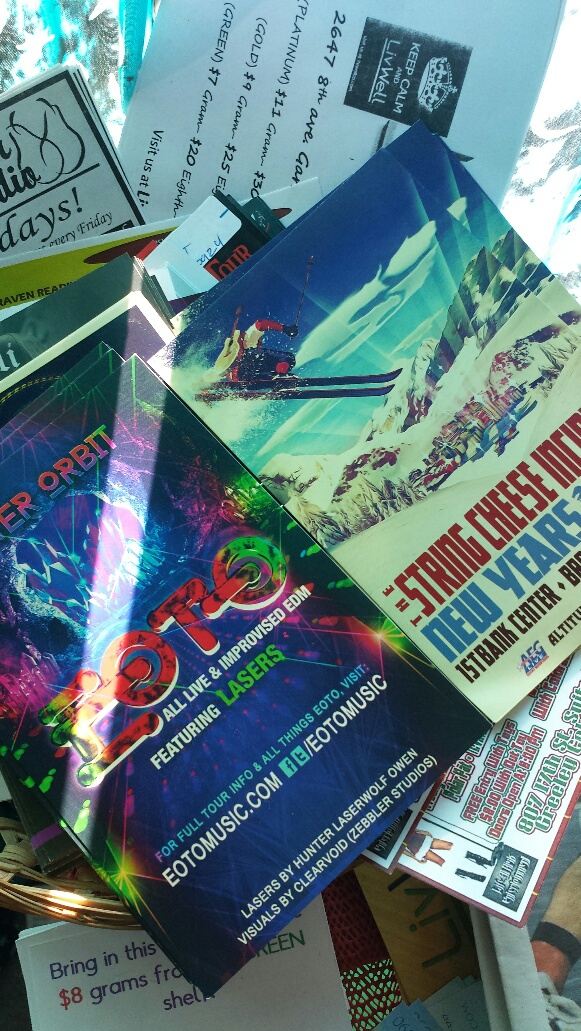The image is a detailed close-up of a stack of assorted books, magazines, and cards, presented in portrait orientation. On the left side, a prominent book with a blue cover and red text reads "EOTO." Below this in white text, it states "All Live and Improvised EDM Featuring Lasers." Further details include, "For a Full Tour Info and All Things EOTO, Visit EOTOMusic.com," with accompanying Facebook and Twitter icons (@EOTOMusic). Additional text at the bottom reads, "Lasers by Hunter Laserwolf Owen" and "Visuals by Clear Void (Zibler Studios)."

In the foreground, there's another book with a blue cover and red print echoing the same EOTO messaging. Slightly to the right, a card features a cartoon of a skier mid-jump with text indicating "The String Cheese Incident New Year's, First Bank Center."

Above these items, the image displays a clutter of overlapping book corners that are not fully legible. There’s also a card displaying "Keep Calm and Live Well" with an address "2647 8th Avenue" and pricing details, "Platinum $11, Gold $9, Green $7."

Lastly, part of a brown woven basket trim peeks in at the bottom left corner, providing a rustic touch to the eclectic assortment.